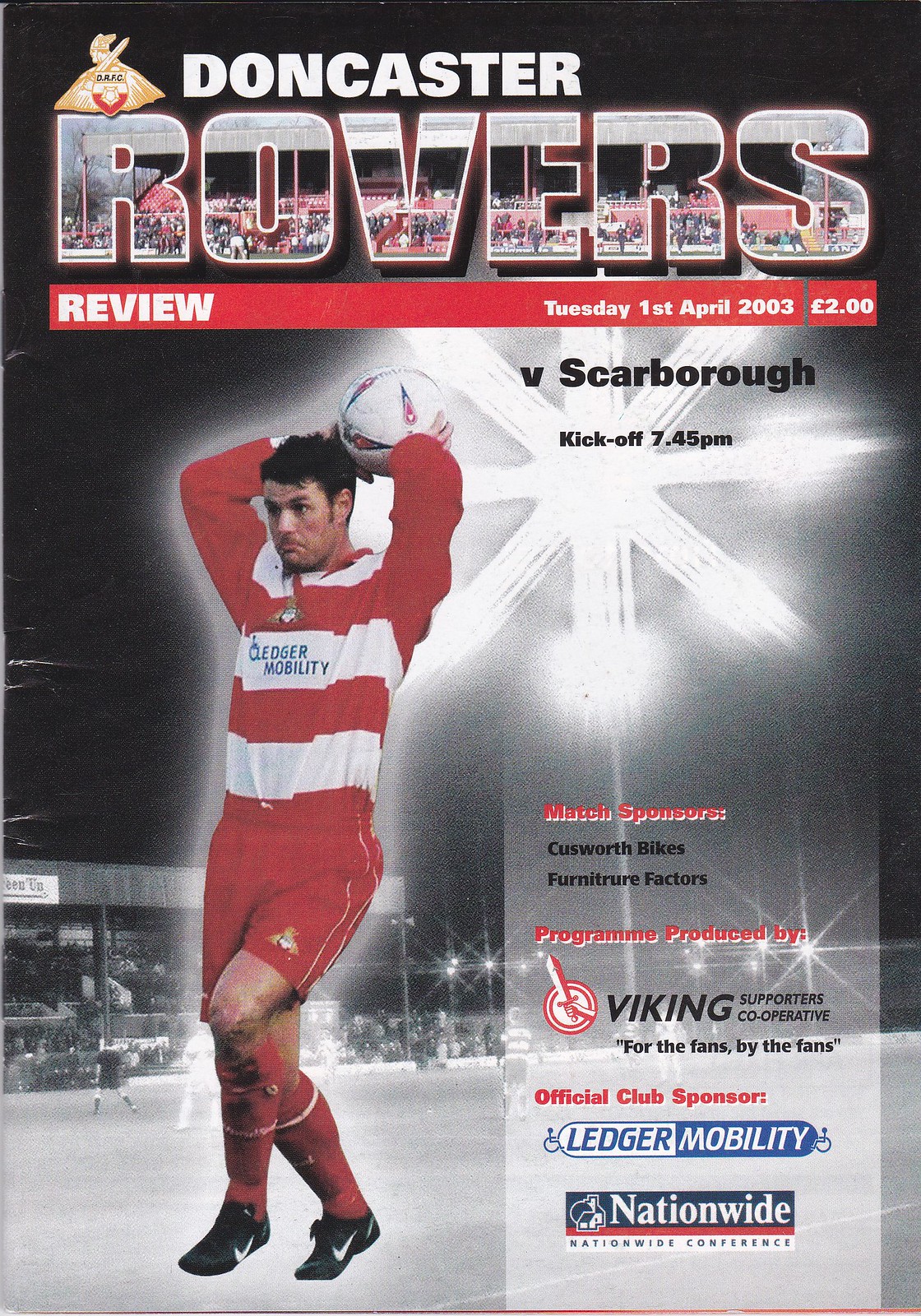This is a program for the Doncaster Rovers football club match against Scarborough, scheduled for Tuesday, 1st April 2003, with a kickoff at 7:45 p.m. The top of the program features the name Doncaster Rovers, with "Doncaster" in plain white text and "Rovers" in bold bubble letters filled with photographs of the spectator stands. Below this, a red background holds white text displaying "Review, Tuesday, 1st April 2003," and the price of £2. The cover also showcases a player poised to throw a soccer ball, dressed in a red and white long-sleeved striped jersey, red shorts, red socks with white stripes at the top, and black shoes. The sponsor Ledger Mobility is visible on his jersey. Background elements include a bright light resembling a snowflake and various sponsor names such as Cussworth Bikes, Furniture Factors, and Nationwide. The program was produced by the Viking Supporters Cooperative.